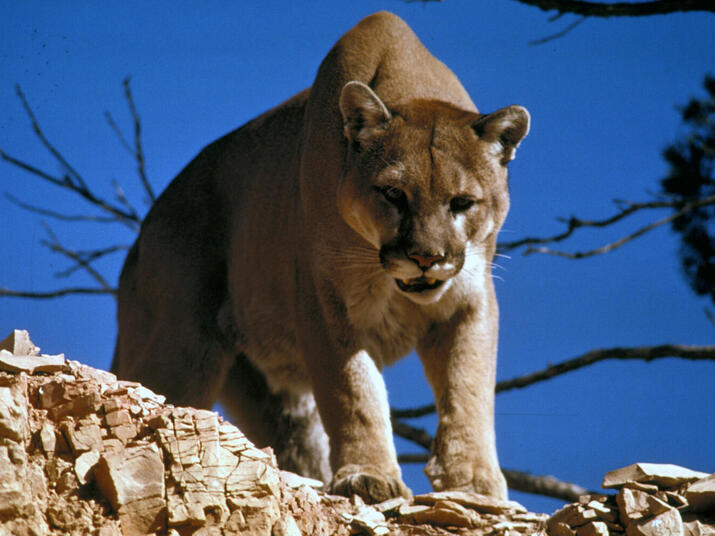This is a detailed and realistic photograph of a mountain lion, also known as a puma, captured in the rugged mountains. The wild cat, exhibiting a soft, sandy-brown coat, is prominently positioned at the center of the image, standing on a craggy outcrop of tan-colored, broken rocks. The mountain lion's powerful build is highlighted with its high-shouldered stance, pointy ears, and big paws. The feline's head is facing slightly downward, showcasing its whiskers and partially bared fangs, giving it an intense and slightly menacing look. The background contrasts sharply with a serene Grecian blue sky, dotted with bare branches, and a darker bush-like shadow on the right side of the frame. The photograph captures the intricate details of the mountain lion's furry coat and expressive features, making it a striking portrait of this majestic creature in its natural habitat.